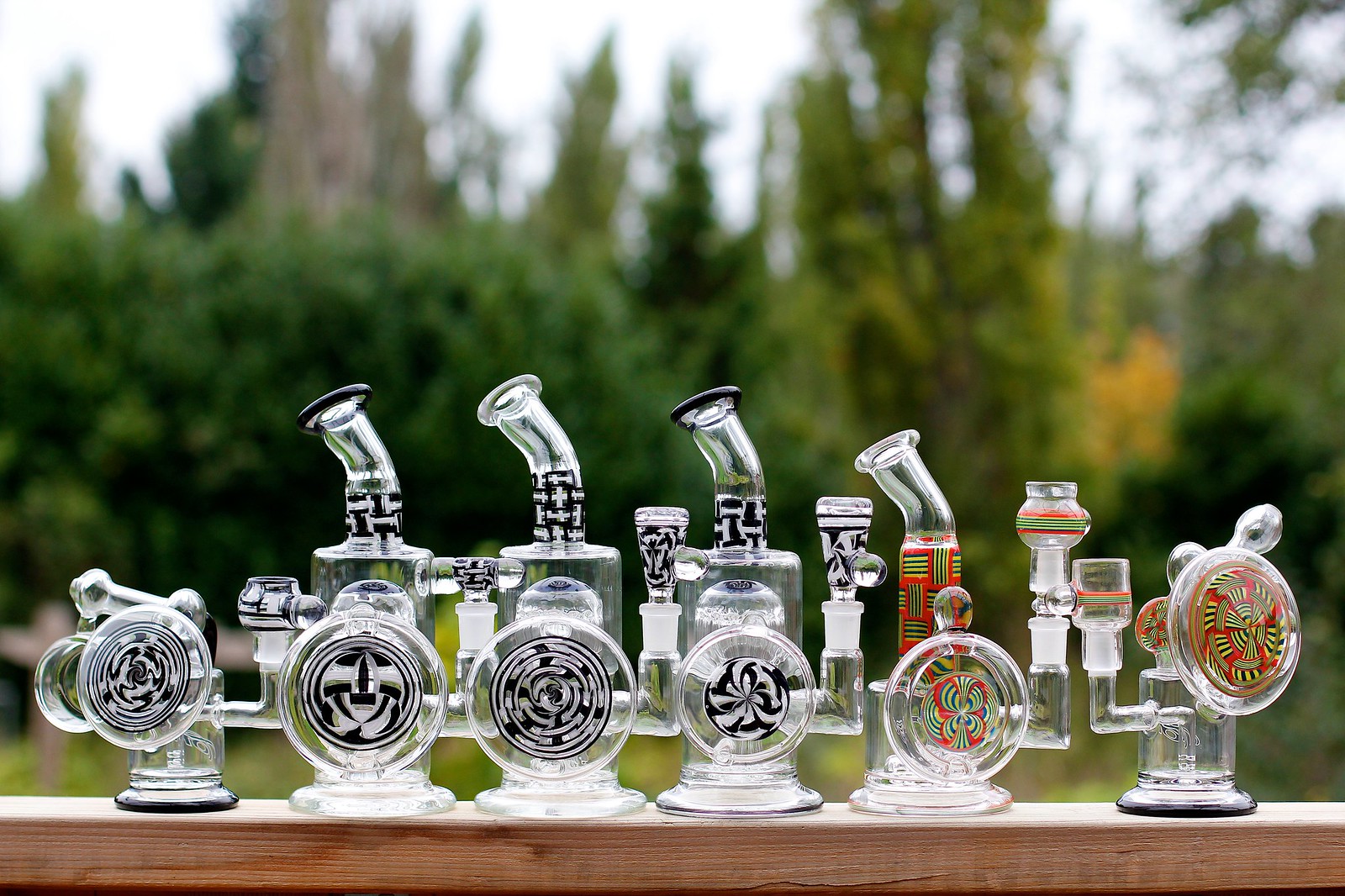This photo captures a collection of six intricately designed glass bongs, carefully lined up on what appears to be the wooden railing of a deck. Each bong features unique artistic elements, with four of them adorned in black and white tribal figures and symbols, while the remaining two showcase vibrant, multi-colored designs, one notably exuding a Rastafarian vibe with red, orange, green, and black hues. The glass bongs possess a sleek structure, with detailed motifs including circular designs and what could be interpreted as Iron Man coils. The image's focus is sharply on the glassware, highlighting their artistic craftsmanship, while the background blurs into a soft scene of greenery, suggesting trees, bushes, and a possibly overcast sky, enhancing the outdoor setting's tranquil ambiance.